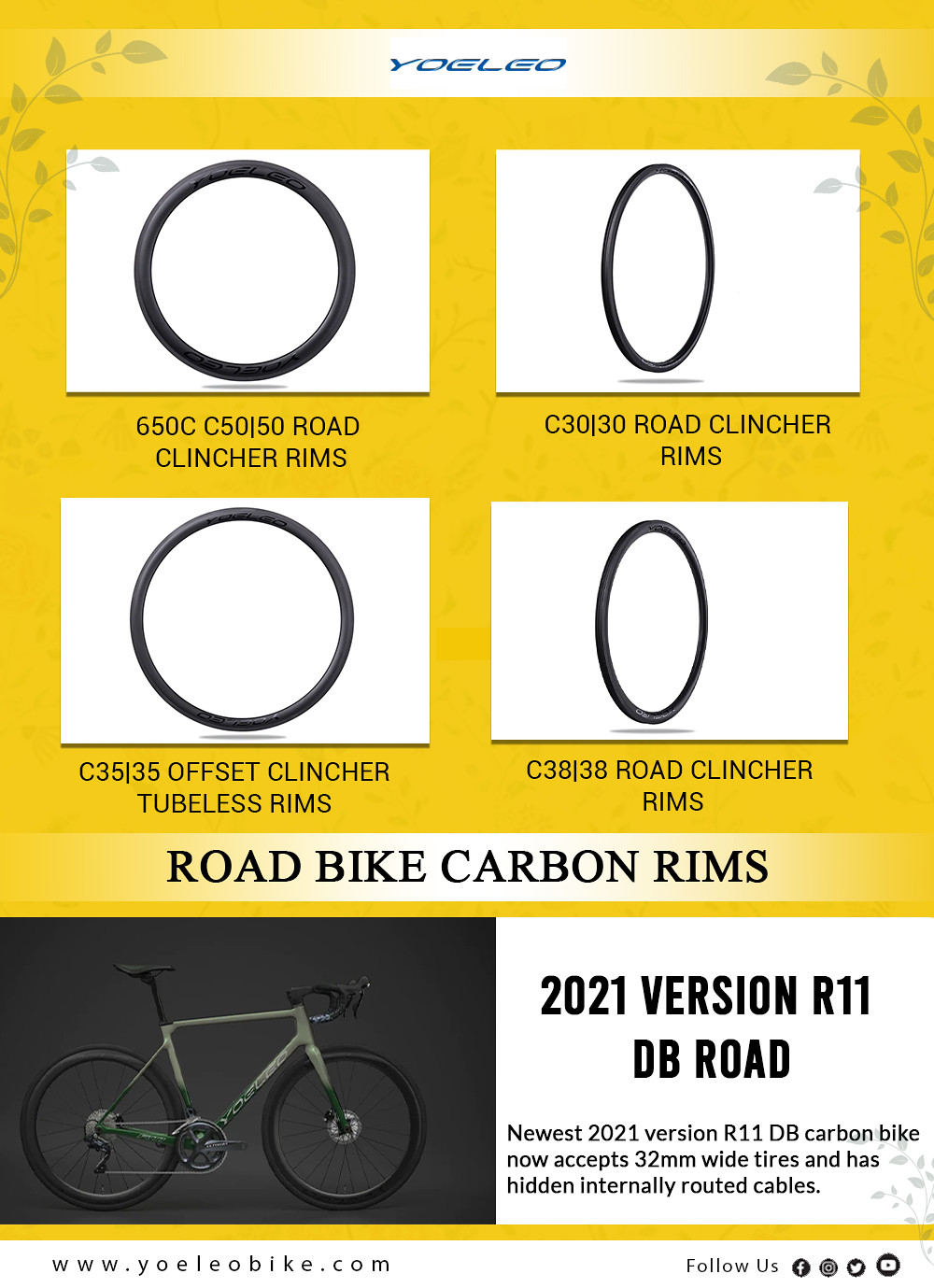This image is an advertisement for Yoeleo's road bike carbon rims and features a poster-like design. The background is yellow, prominently displaying four different types of rims at the top: C5 050 road clincher rims, C30 30 road clincher rims, C35 35 offset clincher tubeless rims, and C38 38 road clincher rims. Each rim is showcased in a clean, white photo. Below the rims, the caption "Road Bike Carbon Rims" is stated, followed by an image of a bike in black and white positioned towards the bottom left. The bike, labeled as the "2021 version R11 DB," highlights its new features, including the ability to accept 32mm wide tires and hidden internally routed cables. The advertisement directs viewers to visit www.yoeleobike.com, with additional social media icons for Facebook, Instagram, Twitter, and YouTube displayed.